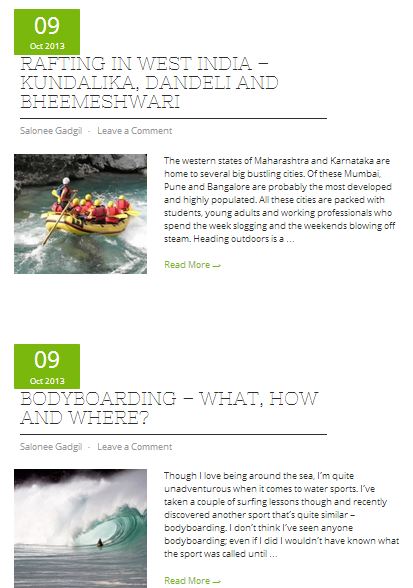Here, presented within a small green rectangle at the top of the image, is the number "09" in bold white text, followed by "OCT 2013" in a smaller white font underneath. Below this, on a white background, the text reads "RAFTING IN WEST INDIA" in capital letters and grey font. The next line specifies "KUNDALIKA, DELHI," followed by another line stating "BHEEMESHWARI," all in the same grey, capitalized style.

Beneath this section, a photograph is placed on the left side, adjacent to a block of text in a faint grey color that narrates:

"The western states of Maharashtra and Karnataka are home to several big bustling cities. Among these, Mumbai, Pune, and Bangalore are probably the most developed and highly populated. All these cities are packed with students, young adults, and working professionals who spend the week slogging and the weekend blowing off steam. Heading outdoors is the..."

The detailed caption and layout provide a structured and informative overview of the context and imagery.